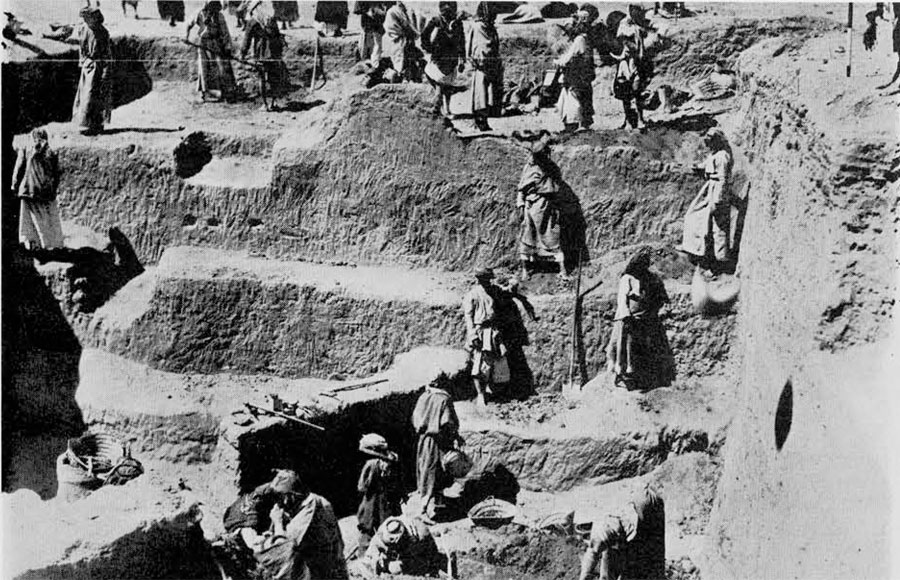This captivating black-and-white photograph is a detailed depiction of an archaeological excavation, likely dating back to the 1800s. The scene is bustling with approximately 25 to 30 individuals, both men and women, actively engaged in delicate digging operations. The dig site, possibly in a Middle Eastern desert given the attire, reveals multiple stepped levels that appear to be the remains of an ancient building being meticulously unearthed from the ground.

At the top of the excavation, workers, some dressed in long robes and head wraps typical of desert wear, and others in more Western attire, including a man in safari clothes and a woman in a skirt and fedora-like hat, stand observing and wielding various tools. The image captures a mix of traditional digging instruments such as shovels, hoes, axes, and hammers, as well as more specialized tools like brooms and surveying equipment, all scattered across the exposed brickwork.

The photograph's heavy shadowing emphasizes the sun’s angle, casting dramatic contrasts across the site and bringing depth to the exposed, ancient structures. Workers are seen at different levels of the excavation, some standing on what appears to be part of a staircase made from partially unearthed walls, while others are deeply concentrated on their tasks, bent over and digging in the dirt at the base. The meticulous work has left visible marks on the walls, evidence of the arduous labor undertaken to reveal the historical treasures hidden within the site.